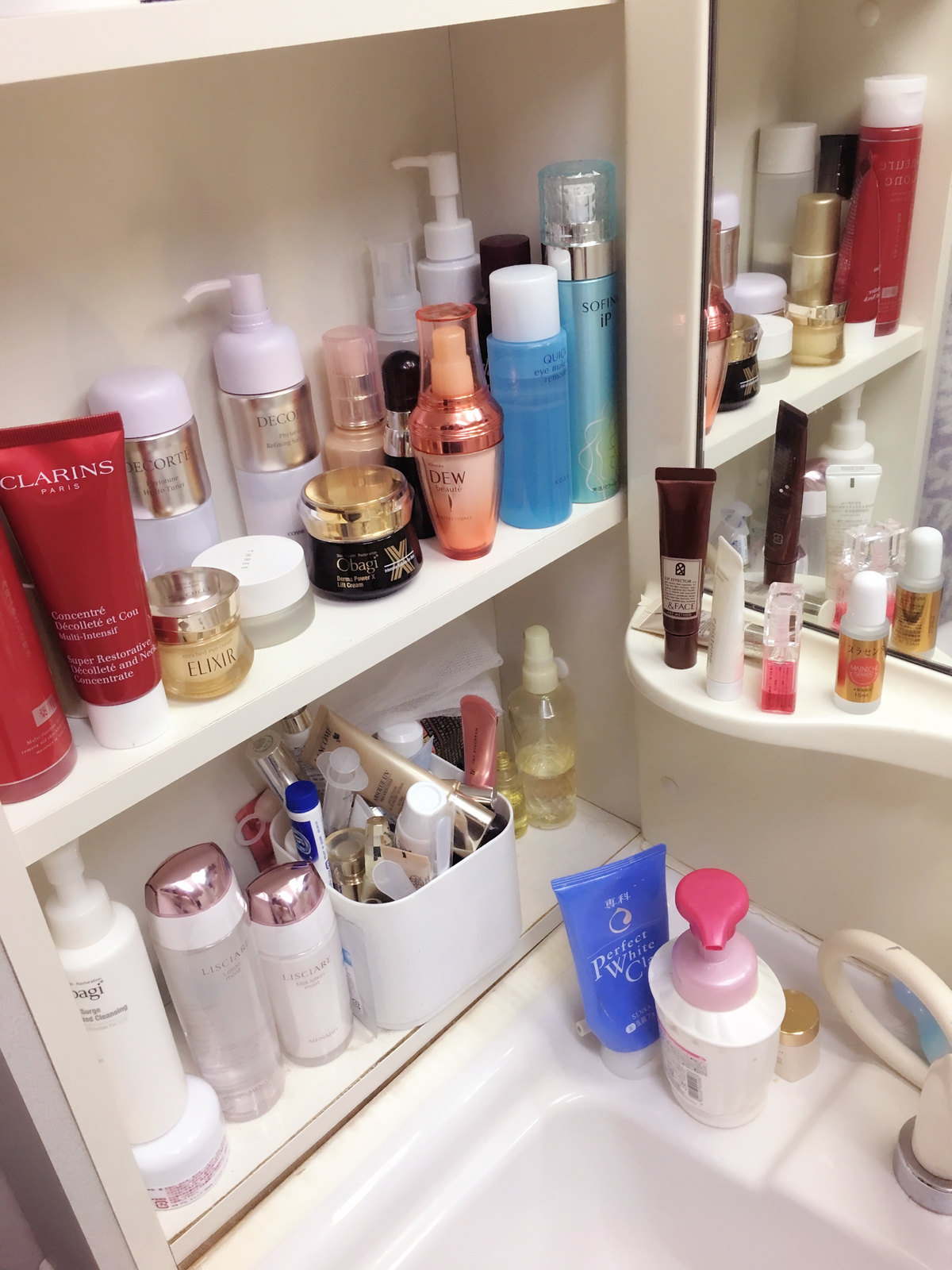The image depicts an open sink area filled with an assortment of toiletry items. Prominently, there are two bottles near the sink – one blue and one white, the white one featuring a light purple and reddish pump. Behind these, a small glass bottle with a gold cap is visible. A tube extends from the bottom right, likely connecting to the sink's tap. 

To the left, white shelving holds numerous bottles. Near the back, pink bottles transition to red, with the red squeeze bottles branded as Clarins from Paris, distinguished by white lettering. Adjacent is a silver-topped gold bottle, followed by more bottles in black and gold hues. Continuing in sequence are shiny pink bottles, one of which appears to be labeled "Dew," and then various blue and light blue bottles. 

In front of a mirror, smaller items such as what appears to be mascara and other women's products are arranged on a white lip extending from the shelf. The mirror itself, framed by a black line, reflects part of the scene. Below, another shelf holds additional bottles and a white container in the middle, housing toothpaste and more toiletries.